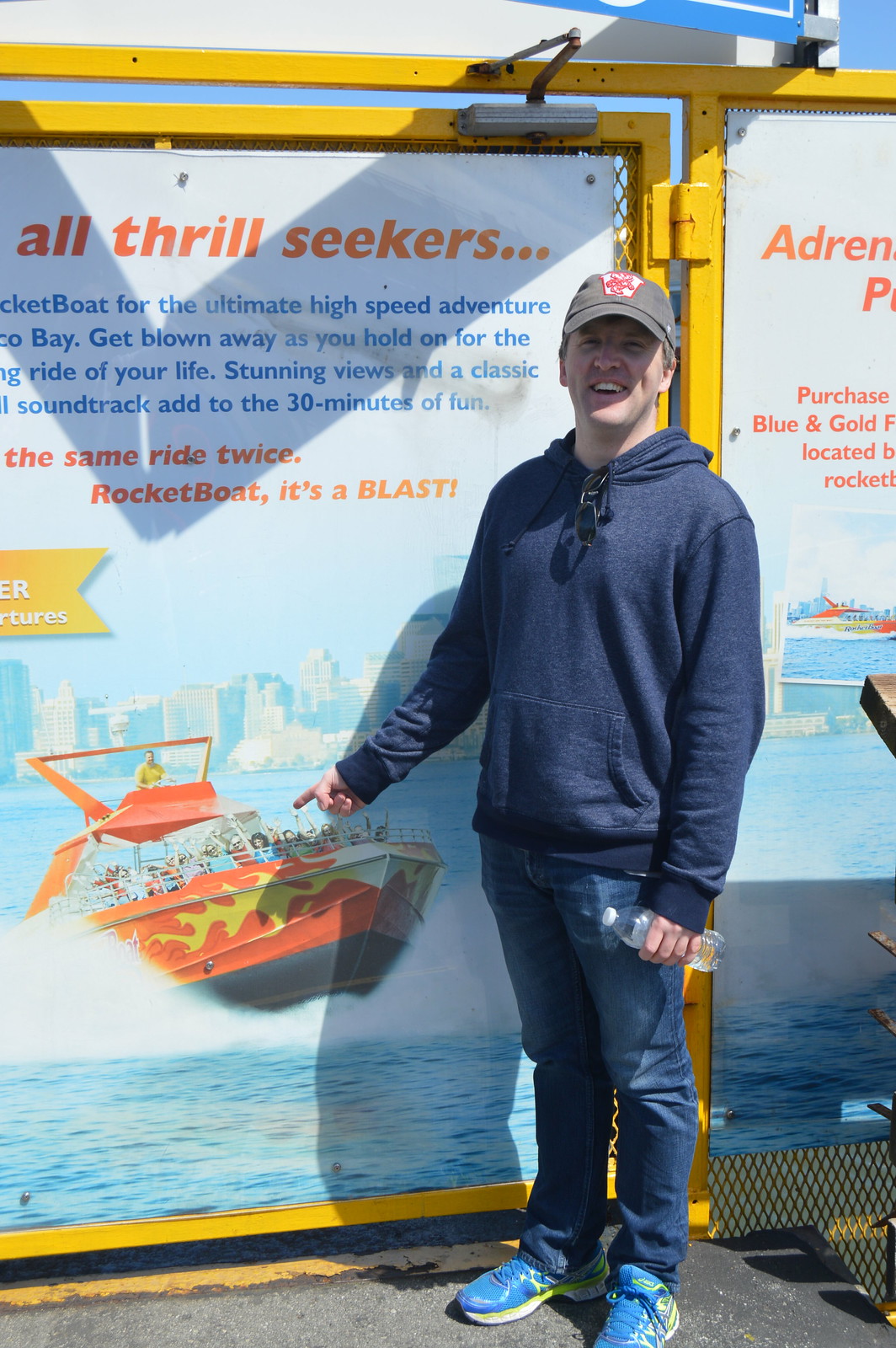In this outdoor image, a man stands on an asphalt surface under bright sunlight, giving the scene vibrant lighting. He is positioned centrally, pointing with his right hand at a large banner showcasing a thrilling boat ride called the "Rocket Boat." The banner reads, "All thrill-seekers: rocket boat, it's a blast, for the ultimate high-speed adventure," and promises stunning views and a classic soundtrack for a thrilling 30-minute experience. The man is casually dressed in a long-sleeved blue sweatshirt, blue jeans, and light blue running shoes with neon yellow accents. He also sports a cap and has sunglasses hanging off the neck of his sweater. In his left hand, he holds a water bottle. The background features posters of boats and shows snippets of blue sky between them, suggesting the scene is set near a harbor or waterway, with some ambiguity about the exact setting.